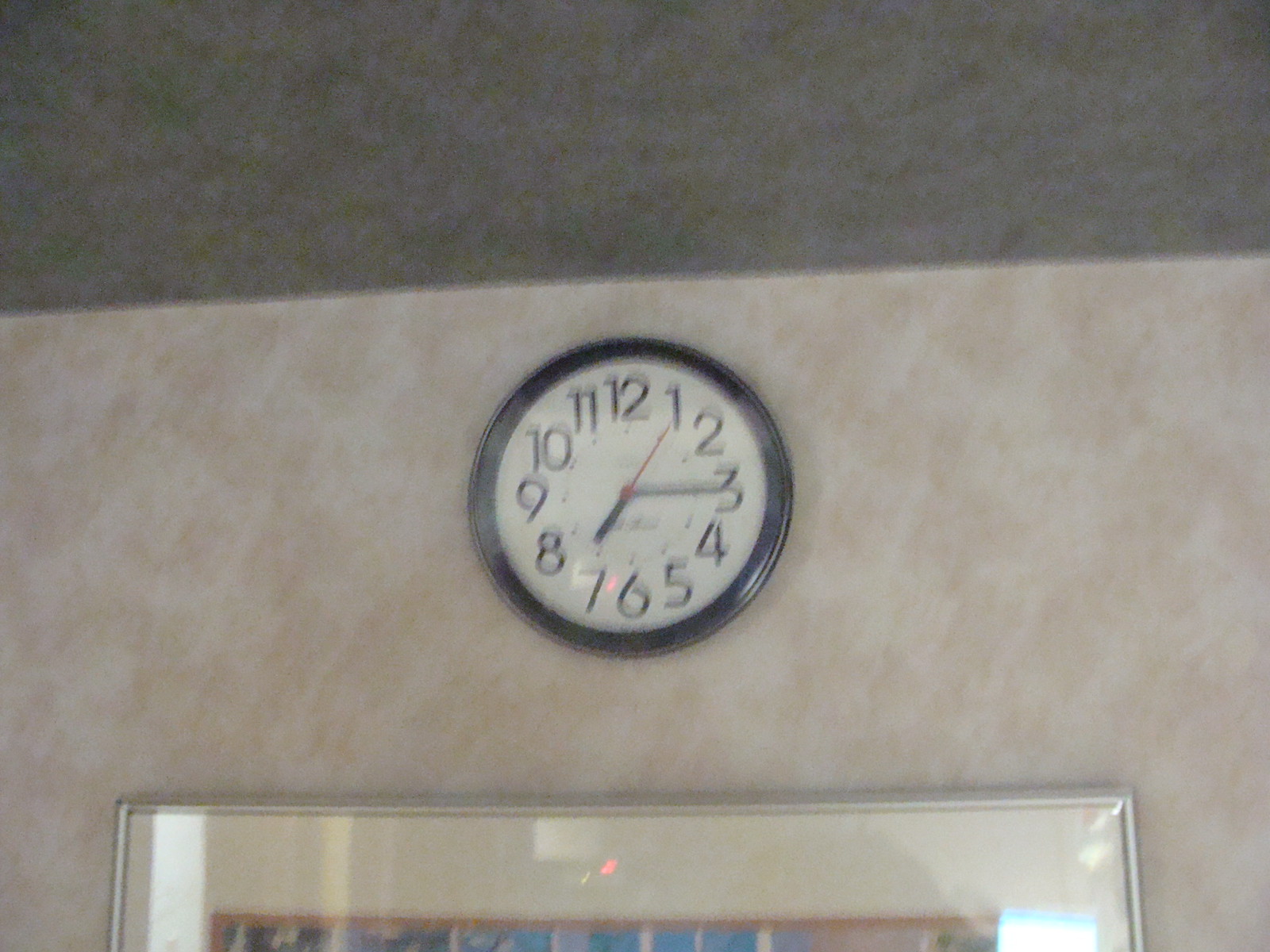This is a blurry, horizontally-oriented photograph of a room featuring a clock mounted on a marble-patterned wall. The wall has a modulated peach and tan color with white marbling, giving it a tie-dyed appearance. The clock is centrally placed, circular, with a black frame that has a slightly shiny finish. The clock's face is white, with modern styled black numbers, and reads 7:15. It has black hour and minute hands and a red second hand currently pointing at the 1. Directly beneath the clock, partially visible, is a silver-framed picture. The frame has a white matting and a medium brown border, with hints of turquoise and orange in the image. The ceiling, slightly darker and similarly patterned as the wall, is visible at the top of the image.